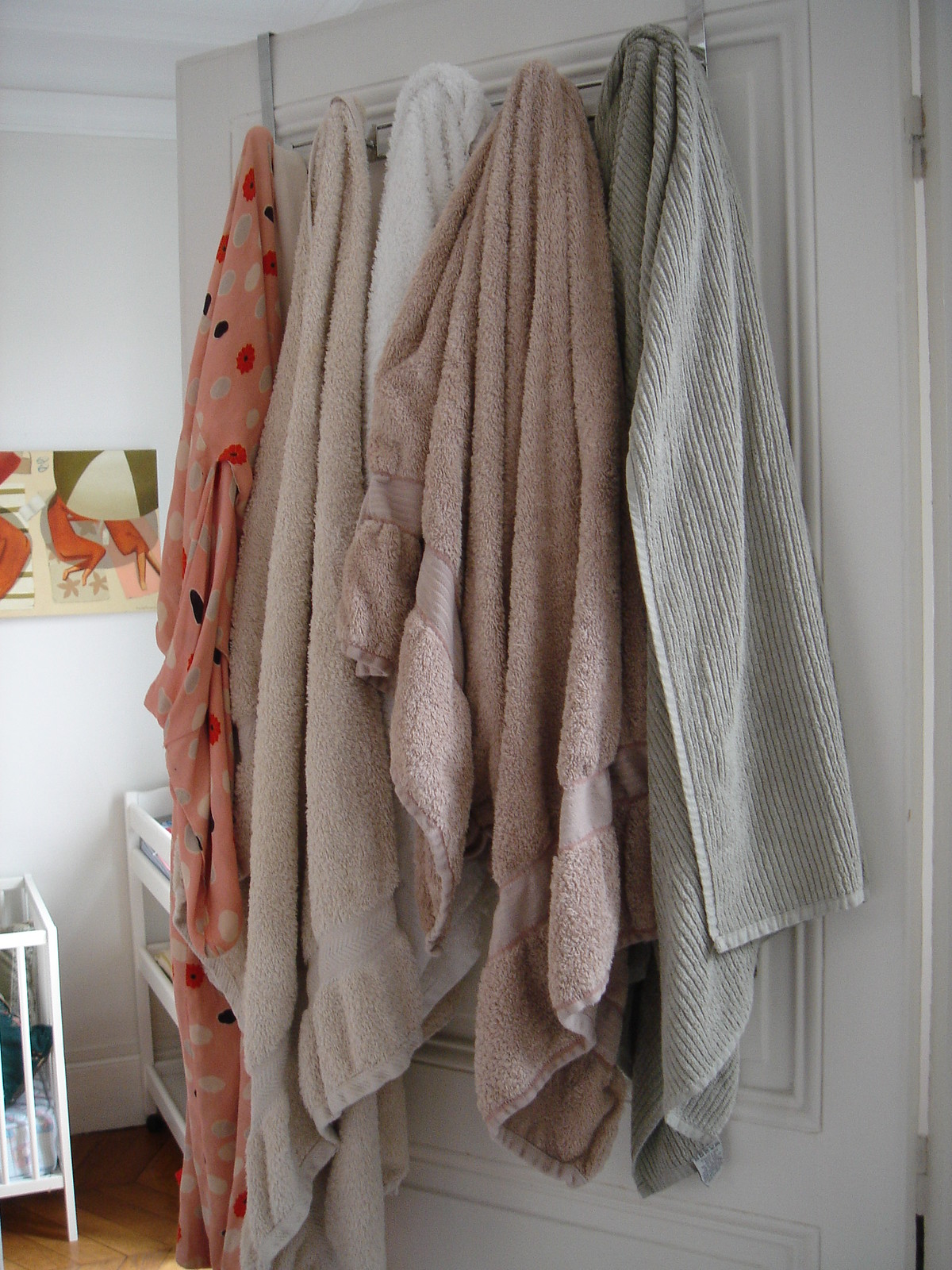This image depicts the interior of a house, focusing on a white door adorned with a series of metal hooks. These hooks are used to hang several towels in a variety of colors and patterns: grey, ribbed grey, light brown, white, pink polka dots (pinkish color with yellow, blue, and red dots), and blush pink. Additionally, a pair of pajamas with blue, red, and white circles also hangs among the towels. In the background, against the white wall, there is a colorful painting featuring hues of orange, green, and a pale white triangle. To the left, there is a crib with white bars, while to the right, a playpen or another crib, also with white bars, can be seen. Further right, a white wooden changing table is placed. The scene is set against natural hardwood floors, creating a cozy and organized nursery or children's room.